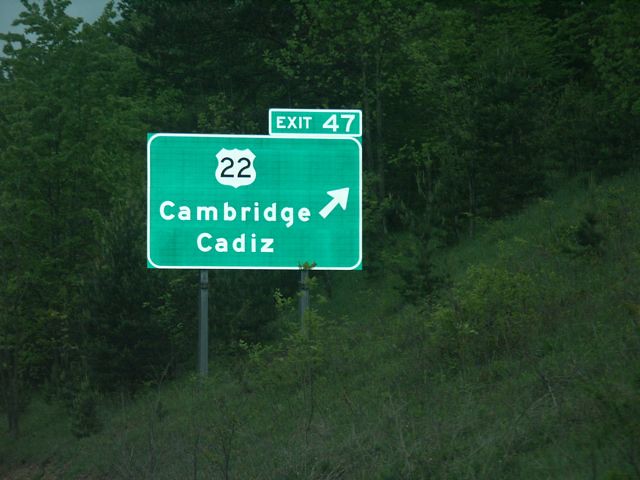The image features a typical freeway sign, primarily green with white trim, standing out vividly against the surrounding landscape. At the top of this main sign is a smaller sign also trimmed in white, displaying "EXIT 47" in bold, uppercase letters. Below this, the larger sign prominently features a shield-shaped symbol with the number "22" in black. Further down, it lists "Cambridge" and "Cadiz" in white text, with a white arrow pointing diagonally upward to the right, indicating the direction to these destinations.

The sign is supported by two slender gray-green poles. The setting is a hilly, grassy area, giving way to a dense forest of trees in the background. In the top-left corner of the image, the sky is visible, appearing slightly gray, adding a muted tone to the picturesque scene.